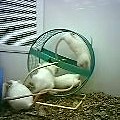This small, blurry, and pixelated square photograph depicts four white mice in an enclosure with a rough textured floor, likely made of wood chips or sawdust. At the center of the image is a green exercise wheel. Two of the mice are inside the wheel, with one positioned upside down as if it has been flipped while running. A third mouse is attempting to join them on the wheel, while the fourth mouse sits nearby, observing. The enclosure has grey walls, and the background includes a vent or window with shutters, along with a faint blue object in the bottom left corner. The image appears to be low resolution, making details difficult to discern.